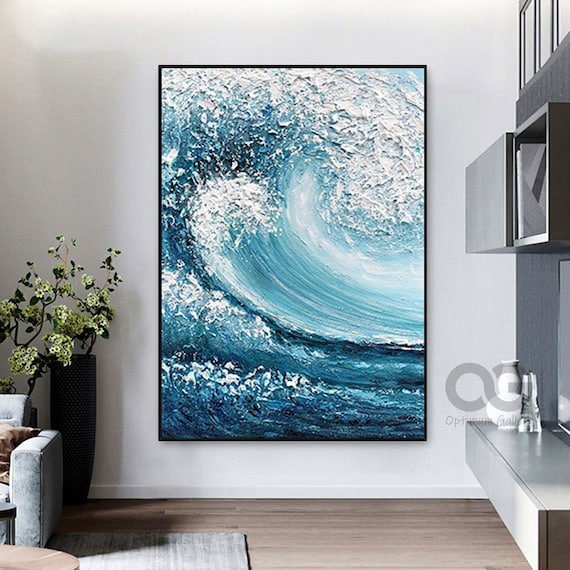The image showcases a living room with a large, vertically rectangular painting of a massive, textured wave as its focal point. The painting, encased in a thin black frame, hangs on a light gray wall. The wave composition is dynamic, with darker blue at the base blending into lighter blue and white froth as it crests towards the right, depicting a vivid, crashing motion. Below the painting, the floor is covered with wood tile, complemented by a tan and white rug.

In the lower left corner, the arm of a light gray sofa or armchair is visible, next to a tall black vase filled with green leaves and white flowers. The bottom right of the image hints at a small table, only partially within the frame. To the right of the painting, a white countertop extends to the floor. Above this counter, gray letters spell out "Optum Gallery" with a large "OG" in the middle, partially obscuring the view of a white drink container. The balanced color palette of light grays, browns, and softer accents adds to the serene and cohesive aesthetic of the room.